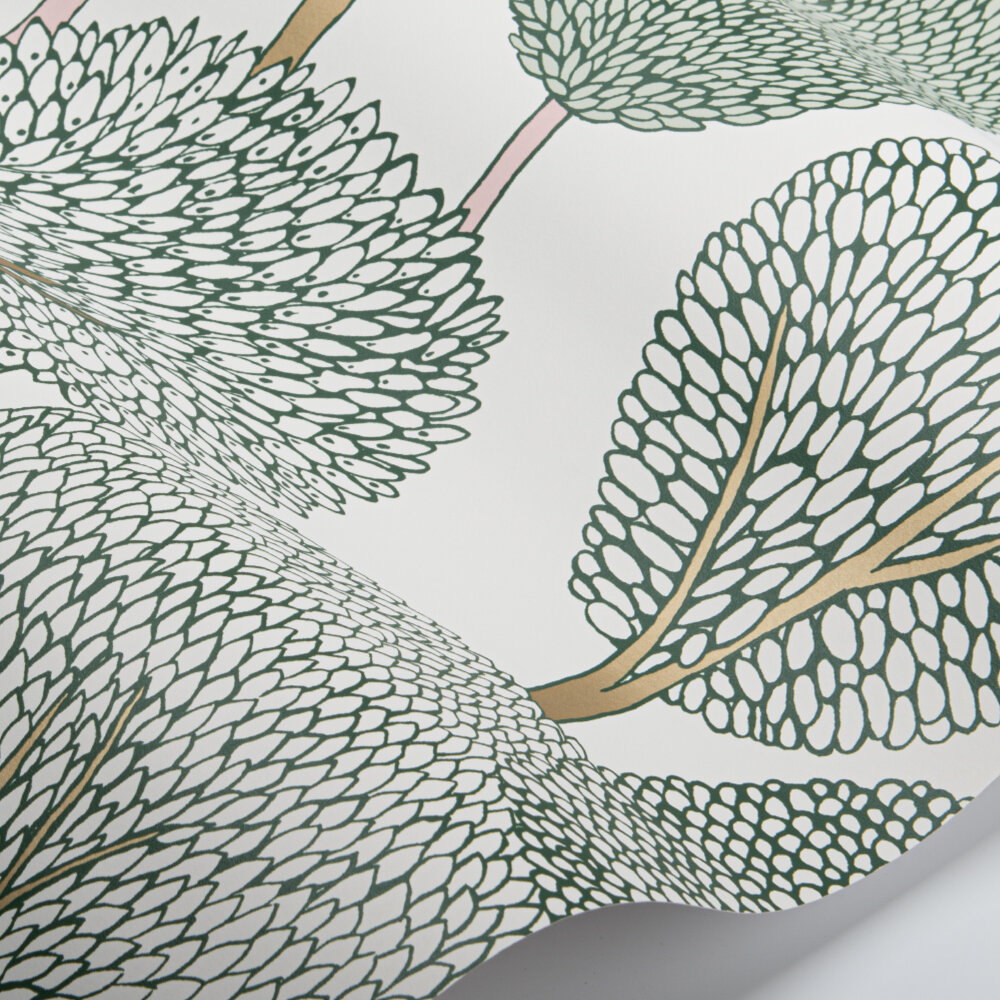This image depicts an intricate drawing on a slightly wavy piece of white paper that casts a shadow on the background. The artwork features a series of distinctive trees rendered in a unique style, where the canopies are composed of ovals nested within ovals, resembling dragon scales or lizard skin. Each tree is different, exhibiting its individuality through variations in color and detail. Some tree trunks are pink, while others are a light brown or golden beige. The foliage primarily appears in shades of green, with certain trees displaying a dark gray to black hue. One tree stands out with its green and oval-shaped leaves, while another is notably dotted. The trees are scattered with large spaces in between, and some extend off the edges of the paper, suggesting their continuity beyond the visible frame. The entire drawing is simple yet artistic, combining straight and curved lines with detailed oval leaves, giving a textured, almost bushy appearance to the branches.